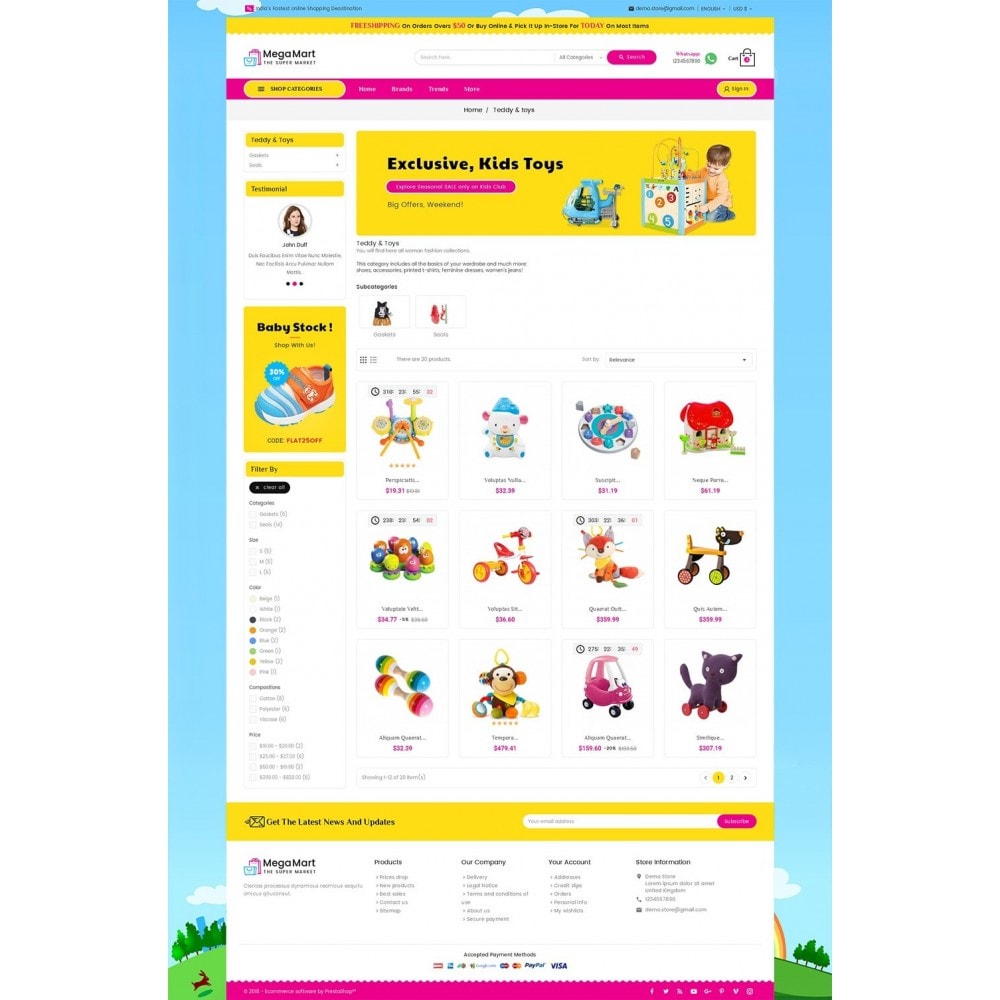The image depicts a colorful, engaging scene from a shopping website, featuring a whimsical and vibrant design. The background is light blue with white clouds and a grassy hill at the bottom, dotted with trees, animals, and a partial rainbow.

The website itself is primarily in shades of yellow, white, and pink. At the top, there's a yellow banner with black and pink accents, although the font is unreadable due to blurriness. Directly above this banner, there is a black sentence, and black submenus are placed above it. Below the banner, a white box possibly displays the company's name "Mega Mart" in black text, with a slightly blurry pink and blue logo next to it. Adjacent to this is a white search box, and right beside it, a pink and white search box. A small green phone icon with a phone number and a black shopping bag icon are also visible.

Descending further, a pink bar adorned with gold and white elements directs the eye downward to a section where products can be sorted. This area features gold, white, and black menus. Below this, there's an image of a woman with two lines of text underneath and an ad for baby products featuring a blue and orange shoe.

Continuing further down, submenus allow sorting by various criteria such as color and ratings. A prominent black banner announces "Exclusive Kids Toys," accompanied by a pink bubble and an image of a little boy dressed in orange, playing with a device that has numerous numbers and a blue toy beside it. Below this banner, there’s a vibrant array of brightly colored toys in shades of pink, orange, yellow, and green. The collection includes:

- A lamb-like creature with a blue cloud on its head
- An insect-like creature in blue, orange, and yellow
- A white, blue, and red play wheel device
- A tan and red mushroom-shaped house
- Blue, orange, yellow, and pink creatures
- A red, yellow, and white tricycle
- A little fox in a yellow sweater
- A walking horse-like toy in black, yellow, and green
- Two rattles in green, yellow, blue, pink, and white
- A brown, orange, and yellow monkey toy
- A pink tricycle
- A black cat toy on red wheels

Further down, another yellow box with a search box is seen, followed by a white section filled with black text and submenus. At the very bottom, there are icons indicating accepted payment methods, including Visa, PayPal, and MasterCard, along with another pink strip finalizing the scene.